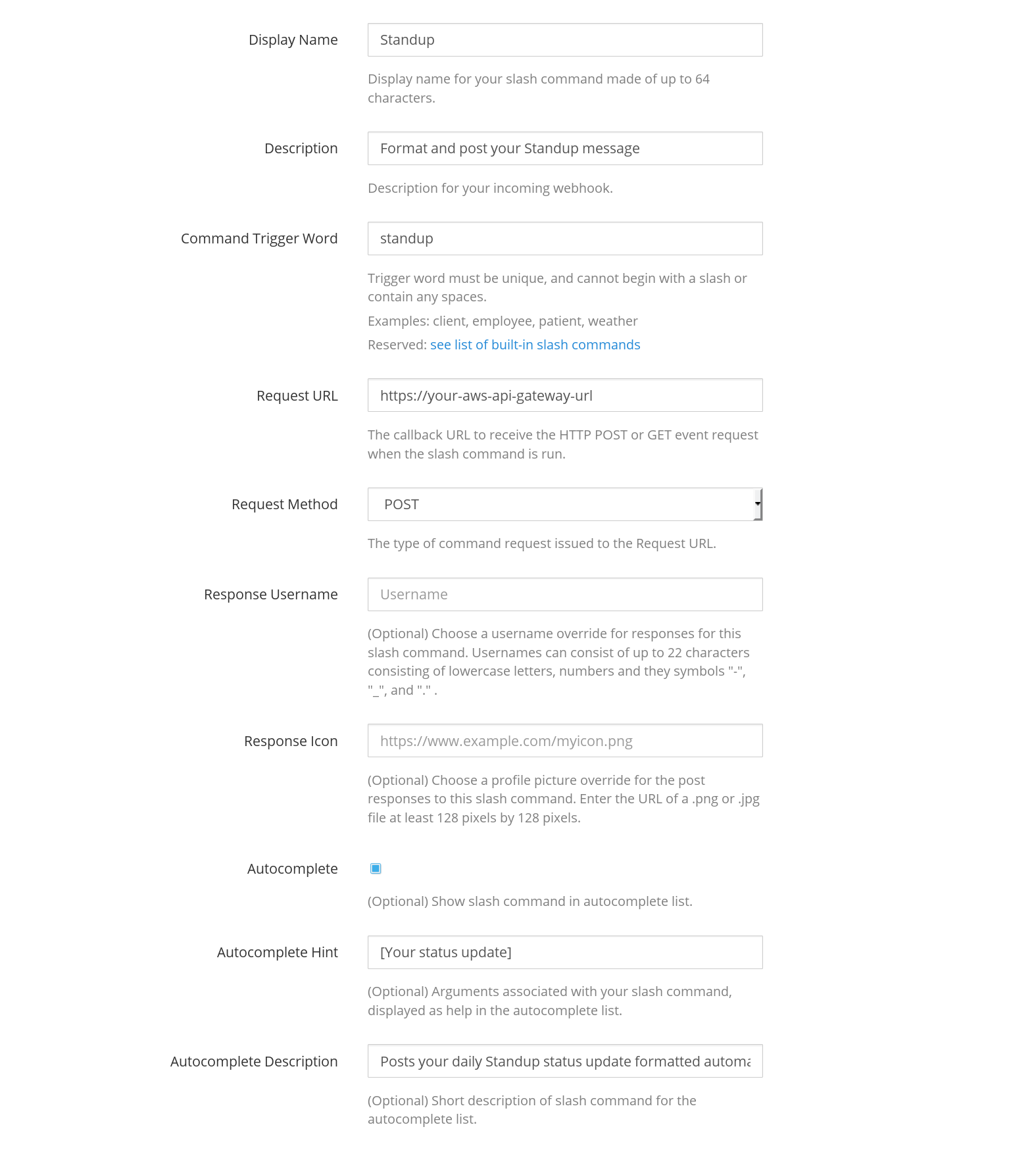The image depicts a structured form interface designed to collect specific information. At the top, there's a field labeled "Display Name" with the text "Stand Up" entered. Below that, a "Description" field contains "Post your stand-up message." 

Next, there's a section labeled "Command Trigger Word" with "stand up" inputted. The "Request URL" field includes a URL, followed by the "Request Method" field which is set to "POST." The "Response Username" field is empty, while the "Response Icon" field has an example URL in it.

An "Autocomplete" button is highlighted in blue, indicating its active status. Below this, there's an empty field for "Autocomplete Hint" with a prompt stating "Your status update." The "Autocomplete Description" reads "Post your daily stand-up status update to format it automatically."

The form consists of nine fields total, each with placeholder text guiding the user on the required input. The background of the page is stark white with black text, making the interface clear and easy to follow.